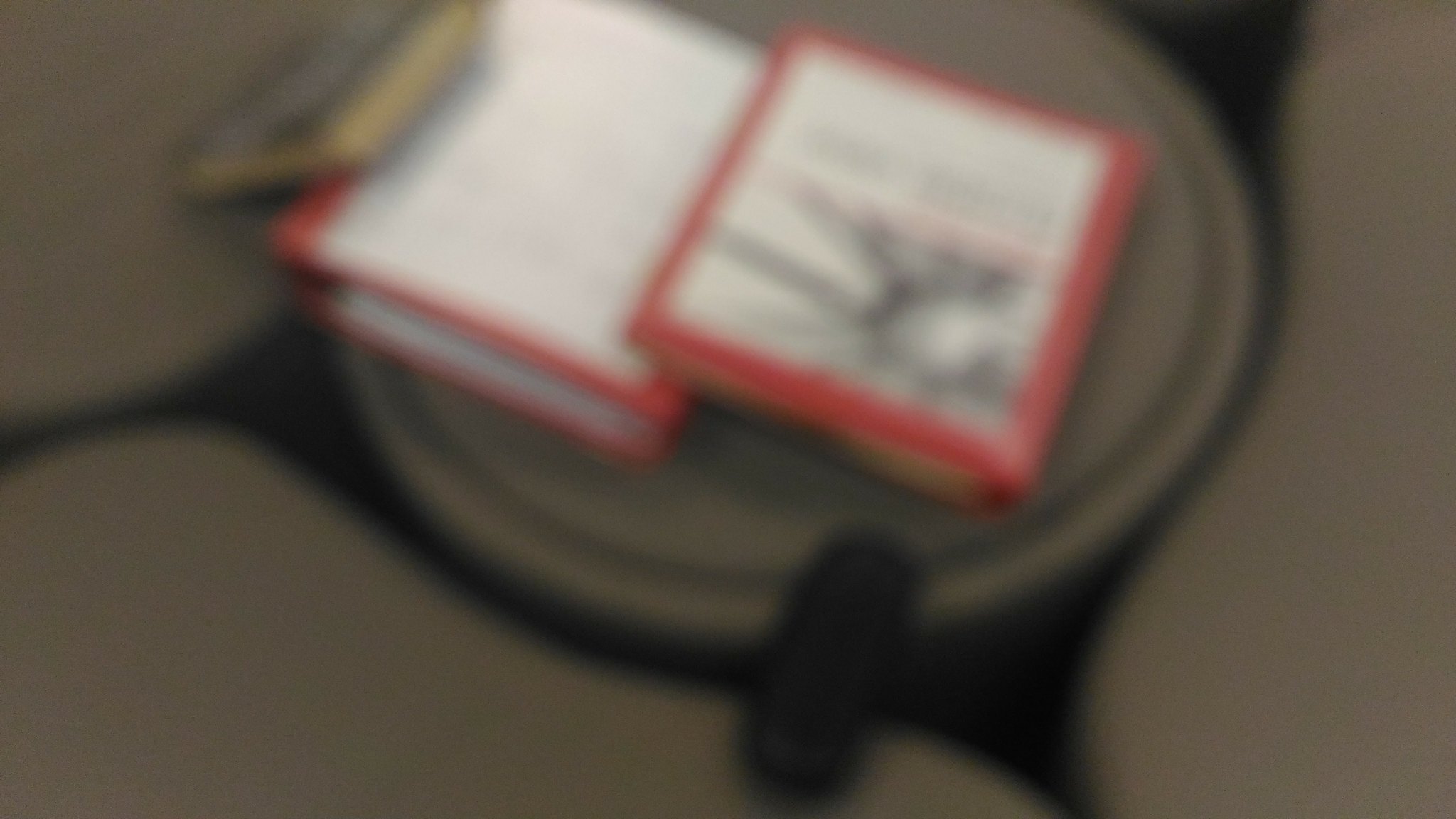A very blurry and out-of-focus image depicting a possible group of four books, three of which have white covers with red trim around their edges. The fourth book stands out with a yellow trim. The background, also quite indistinct, seems to feature some type of cushions—perhaps seat cushions. Two of the books are neatly stacked together, while the book with the yellow trim is slightly tilted, leaning from the left against the stacked pair. Another book on the right side mirrors this arrangement by leaning on the two stacked books from that direction.